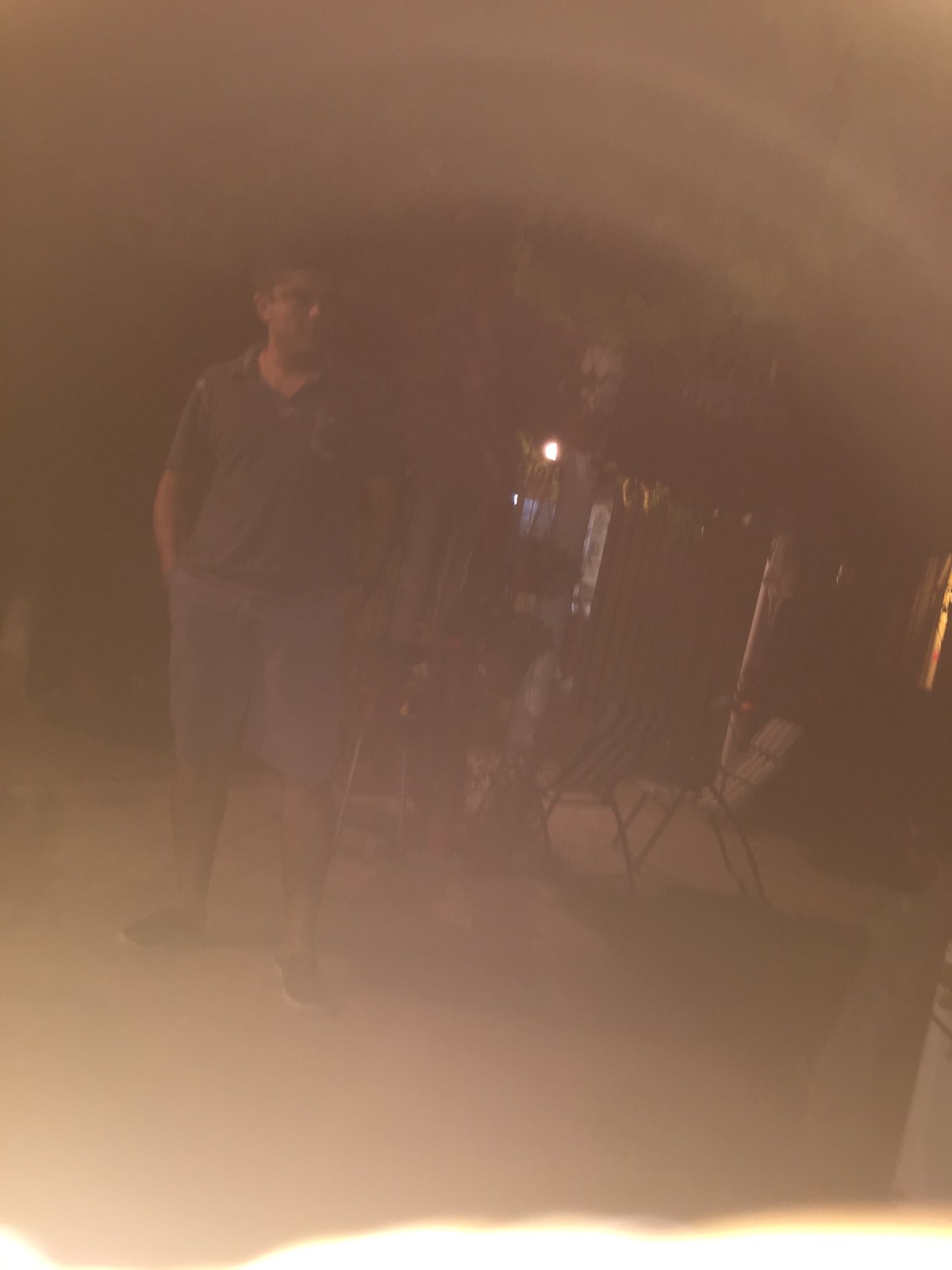In this dimly lit photograph, a man is standing outside on a patio with a concrete surface beneath his feet. He is dressed in blue shorts and a short-sleeved polo shirt that appears to be either black or dark gray. His footwear consists of black tennis shoes with white soles. With his hands casually tucked into his pockets, the man, who has short dark hair and glasses, gazes off to the side. Behind him, a couple of striped folding chairs, featuring a pattern of white and dark-colored canvas, are visible. The background is quite murky, making it difficult to discern further details, though there appears to be an archway or perhaps a reflection, contributing to the overall mysterious atmosphere of the scene.